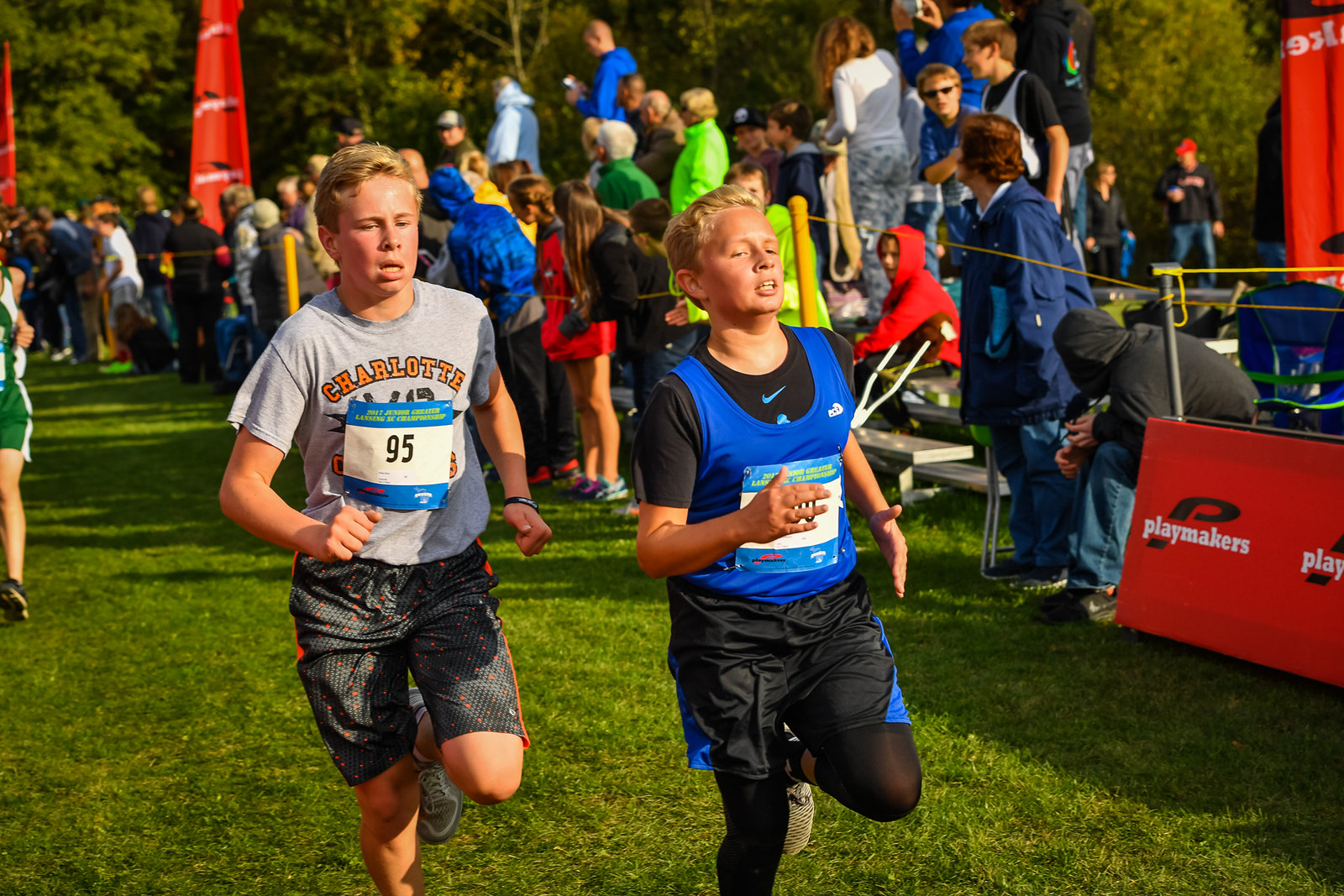The image depicts an outdoor running marathon featuring two blonde boys, both appearing to be in close competition. The boy on the left, wearing a gray t-shirt with the number 95 and gray basketball shorts with orange polka dots, is paired with gray shoes. The boy on the right, slightly ahead, dons a blue sports tank top over a black undershirt, black basketball shorts, long black tights, and has his arms in a running position, obscuring his race number. They are sprinting across very green grass, with a large audience in the background, some standing on tables to get a better view. On the right side of the frame, there's an orange desk with "Playmakers" written in white text, and to the far left, two orange flags are visible, indicating the race area.